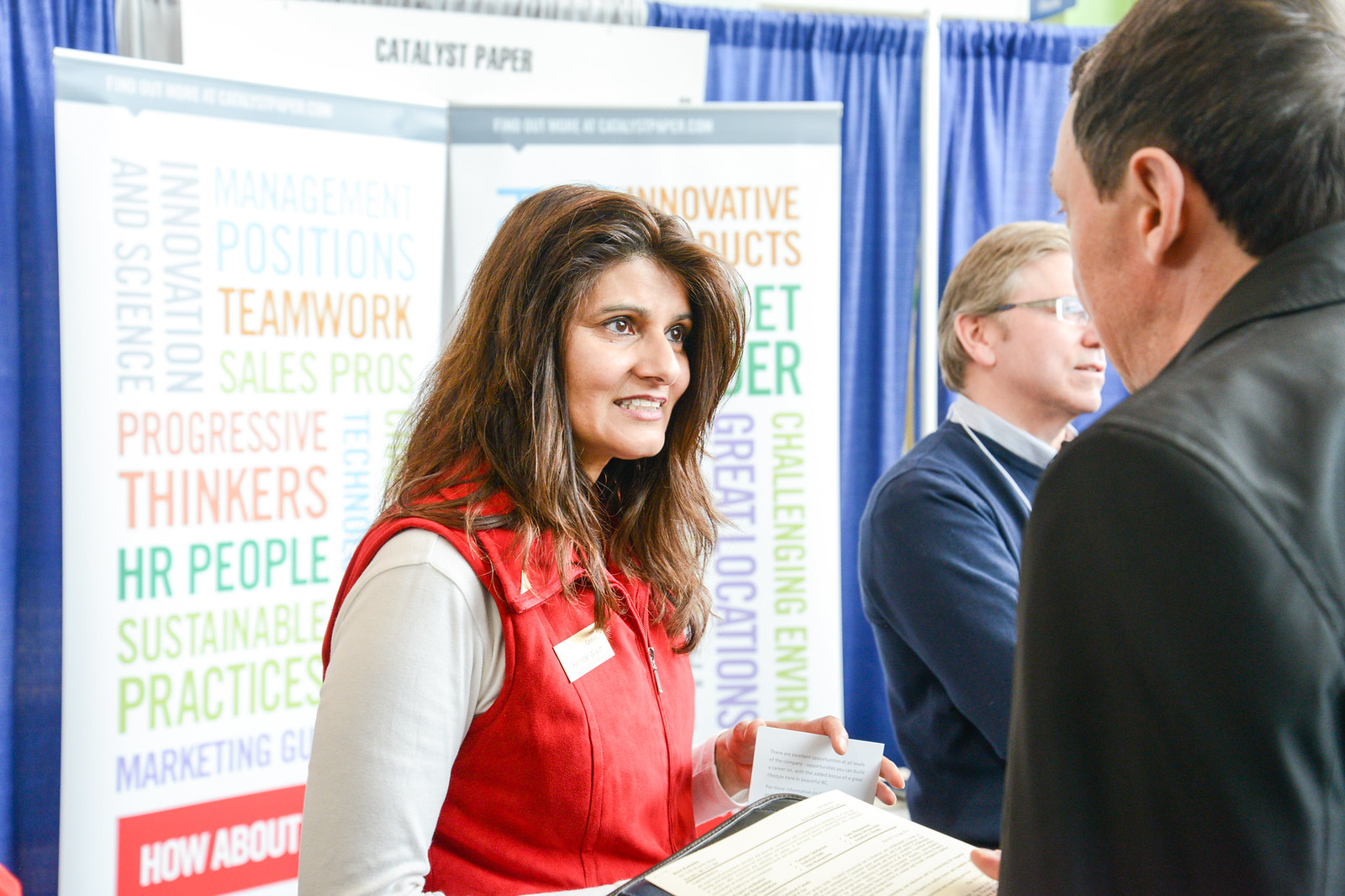In the image, a woman with brown hair, wearing a red jacket or vest over a white long-sleeve shirt and a name tag, stands at a booth during what appears to be a conference or career fair. She is smiling and interacting with a man to her right, who is partially visible from the rear left side, wearing a black leather jacket and holding what seems to be a resume or a folder. The woman holds a brochure or business card in her left hand. They stand in front of a blue curtain, with a banner in the background featuring words like "positions," "management," "teamwork," "sales force," "progressive thinkers," "HR people," "sustainable practices," "innovation," and "science." Another person, partially visible, appears in the background.